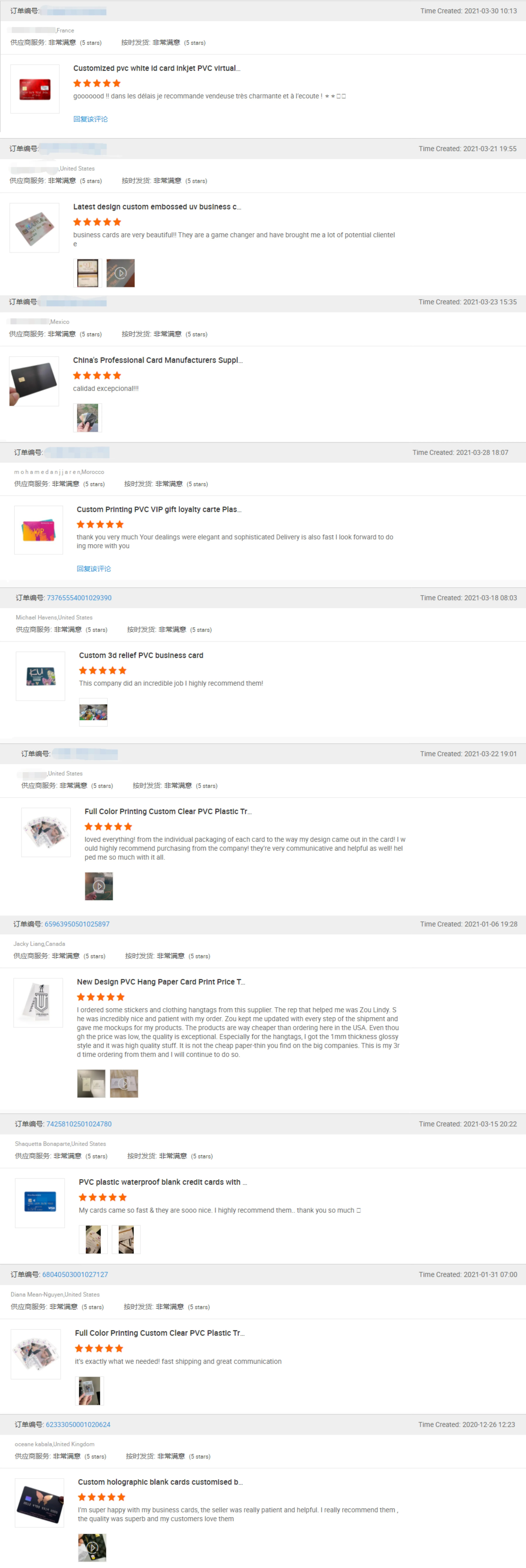**Descriptive Caption:**

The screenshot is a comprehensive, detailed capture of various items listed in what appears to be an online store or review platform, featuring predominantly Far Eastern text (likely Chinese) alongside English descriptions and star ratings for different products. The interface shows a gray banner at the top with Far Eastern text on the left and blue, blocked-out text beside it. The banner on the right mentions "Time Created."

1. **Item 1:**
   - **Timestamp:** 2021-03-30, 10:13
   - **Location:** France
   - **Rating:** Five stars (repeated twice in Far Eastern text)
   - **Product Description:** Customized PVC White ID Card, Inkjet PVC Virtual... 
   - **Review:** "Good!! Donne les délais, je recommande l'industrie charmante et la rectité."
   - **Visuals:** A credit card image

2. **Item 2:**
   - **Timestamp:** 2021-03-21, 19:55
   - **Location:** United States
   - **Rating:** Five stars (repeated twice in Far Eastern text)
   - **Product Description:** Latest Design, Custom Embossed UV Business C...
   - **Review:** "Business cards are very beautiful. They are a game-changer and have brought me a lot of potential clientele."
   - **Visuals:** A tie-dyed card image and a business card displayed front and back.

3. **Item 3:**
   - **Timestamp:** 2021-03-23, 15:35
   - **Location:** Mexico
   - **Rating:** Five stars (repeated twice in Far Eastern text)
   - **Product Description:** China's Professional Card Manufacturers, subplot...
   - **Review:** "Caledon Exceptional!!!"
   - **Visuals:** A black credit card, and an image of someone fanning out several cards like a deck.

4. **Item 4:**
   - **Timestamp:** 2021-03-28, 18:07
   - **Location:** Morocco
   - **Rating:** Five stars (repeated twice in Far Eastern text)
   - **Product Description:** Custom Printing PVC VIP Gift Loyalty Cart...
   - **Review:** "Thank you very much. Your dealings were elegant and sophisticated. Delivery is also fast. I look forward to doing more with you."
   - **Visuals:** A pink and orange VIP card.

5. **Item 5:**
   - **Timestamp:** 2021-03-18, 08:03
   - **Location:** United States
   - **Rating:** Five stars (repeated twice in Far Eastern text)
   - **Product Description:** Custom 3D Relief PVC Business Card
   - **Review:** "This company did an incredible job. I highly recommend them!"
   - **Visuals:** A card with "KU" in large white letters and flower bouquet images.

6. **Item 6:**
   - **Timestamp:** 2021-03-22, 19:01
   - **Location:** United States
   - **Rating:** Five stars (repeated twice in Far Eastern text)
   - **Product Description:** Full color printing, custom clear PVC plastic TR...
   - **Review:** "Loved everything! From the individual packaging of each card to the way my design came out in the card. I would highly recommend purchasing from the company. They are very communicative and helpful as well. Helped me so much with it all."
   - **Visuals:** A fan of business cards with a visible face on the top card.

7. **Item 7:**
   - **Timestamp:** 2021-01-06, 19:28
   - **Location:** Canada
   - **Rating:** Five stars (repeated twice in Far Eastern text)
   - **Product Description:** New design PVC hang paper card, print price T...
   - **Review:** "I ordered some stickers and clothing hang tags from a supplier. The rep that helped me was Zao Lindy. She was incredibly nice and patient with my orders. Zao kept me updated with every step of the shipment and gave me mock-ups for my products. The products are way cheaper than ordering here in the USA. Even though the price was low, the quality is exceptional, especially for the hang tags. I got the one millimeter thickness, glossy style, and it was high-quality stuff. This is my third time ordering from them, and I will continue to do so."
   - **Visuals:** A white card with a sword, business cards, and a video.

8. **Item 8:**
   - **Timestamp:** 2021-03-15, 20:22
   - **Location:** United States
   - **Rating:** Five stars (repeated twice in Far Eastern text)
   - **Product Description:** PVC plastic waterproof blank credit cards with...
   - **Review:** "My cards came so fast and they are so nice. I highly recommend them. Thank you so much."
   - **Visuals:** Pictures of a blue Visa card.

9. **Item 9:**
   - **Timestamp:** 2021-01-31, 07:00
   - **Location:** United States
   - **Rating:** Five stars (repeated twice in Far Eastern text)
   - **Product Description:** Full color printing, custom clear PVC plastic TR...
   - **Review:** "It's exactly what we needed, fast shipping and great communication."
   - **Visuals:** A card held with both thumbs visible.

10. **Item 10:**
    - **Timestamp:** 2020-12-26, 12:23
    - **Location:** United Kingdom
    - **Rating:** Five stars (repeated twice in Far Eastern text)
    - **Product Description:** Custom holographic blank cards, custom B...
    - **Review:** "I'm super happy with my business cards. The seller was really patient and helpful. I really recommend them. The quality was superb and my customers love them."
    - **Visuals:** A black credit card with a multicolored butterfly and a video.